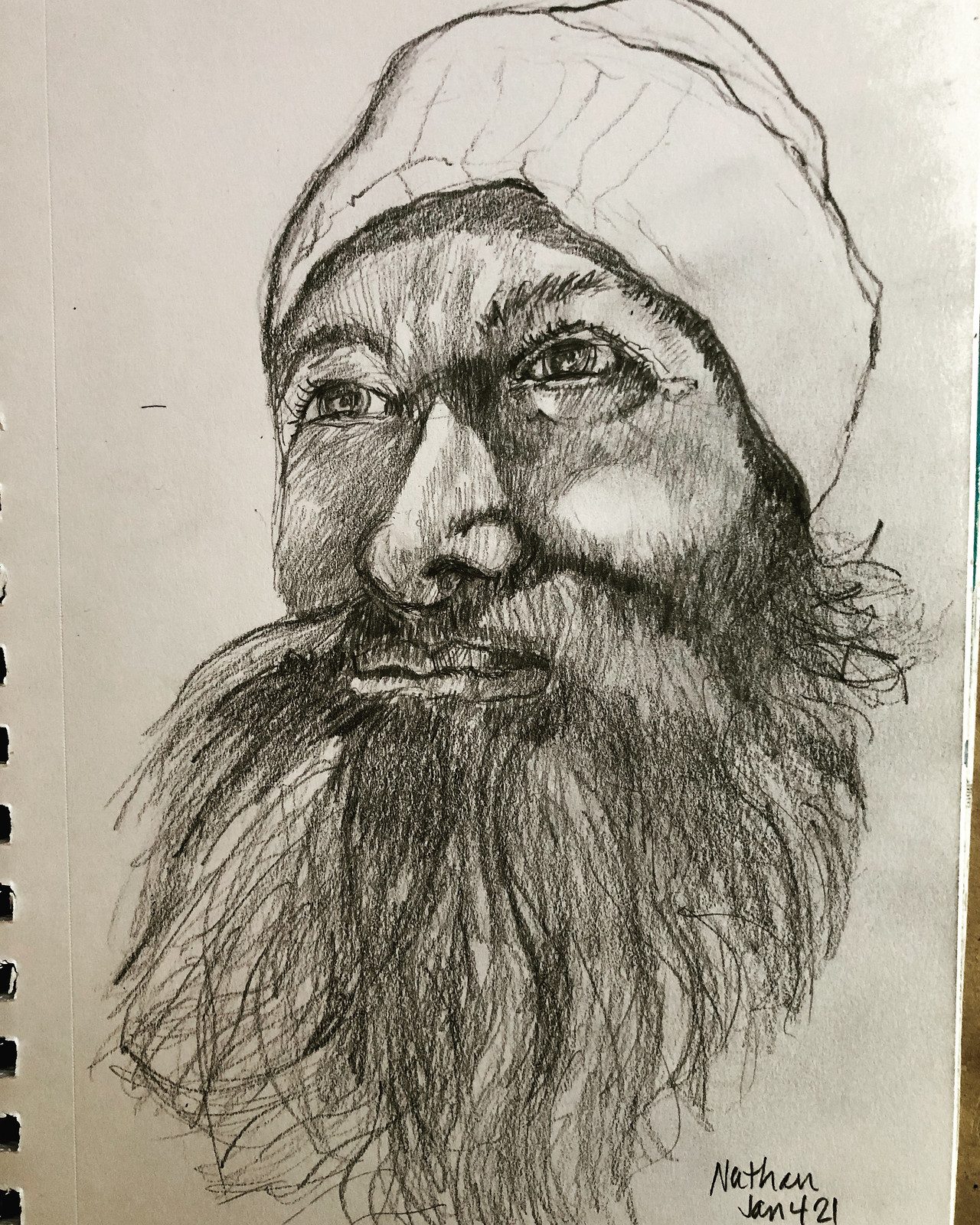This detailed pencil sketch captures the visage of a man, rendered meticulously on a sketchbook that rests on a subtly visible brown surface. The man's face is oriented slightly to the left, showcasing remarkable pencil shading that defines his features. He sports a long, scraggly beard and a matching mustache, both depicted with fine, intricate lines. His lips are clearly visible, adding to the lifelike quality of the portrait. The man is adorned in a stocking hat, illustrated with penciled details that depict its folds and texture, making it appear completely white. Edges of the sketchbook frame the drawing, hinting at the surrounding surface. The artwork is signed at the bottom, reading "Nathan Jan 421," indicating the artist and date of creation.